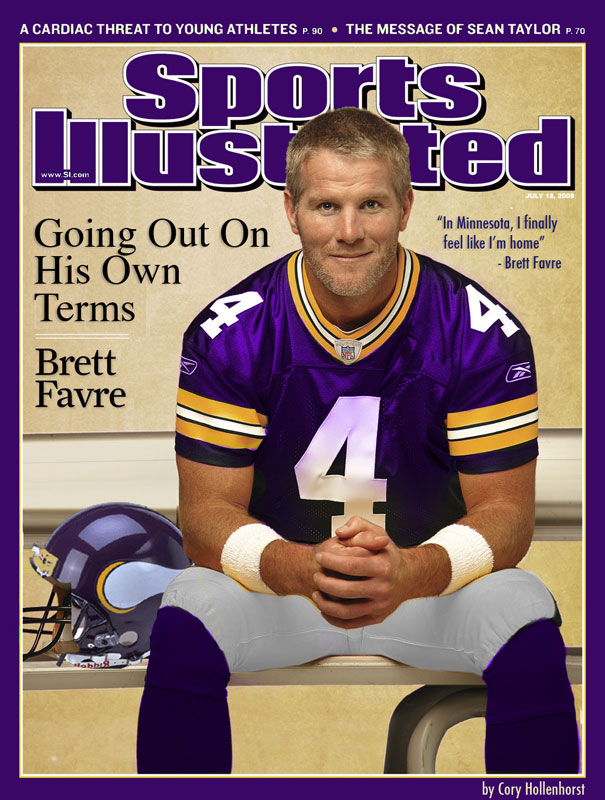This is a detailed description of a Sports Illustrated magazine cover featuring Brett Favre during his tenure with the Minnesota Vikings. The cover itself is predominantly purple, with text at the top reading "A Cardiac Threat to Young Athletes, The Message of Sean Taylor" in white. The Sports Illustrated logo is displayed in purple. Centered on the cover, Brett Favre is depicted wearing his iconic Vikings uniform, featuring yellow stripes on the sleeves, a white number four, and the Reebok logo. He is positioned slightly to the right, sitting with his helmet by his kneecap on his left side. Favre is dressed in white tights and purple stockings. In blue text, a quote attributed to Favre reads, "In Minnesota, I finally feel like I'm home." The bottom right corner credits Corey Hollenhorst. The color scheme of the cover includes purple, white, yellow, black, tan, and beige. Additional text cites page references: "A Cardiac Threat to Young Athletes" on page 90 and "The Message of Sean Taylor" on page 70. The overall composition emphasizes the theme of Favre's personal journey and resolution to play for the Minnesota Vikings.